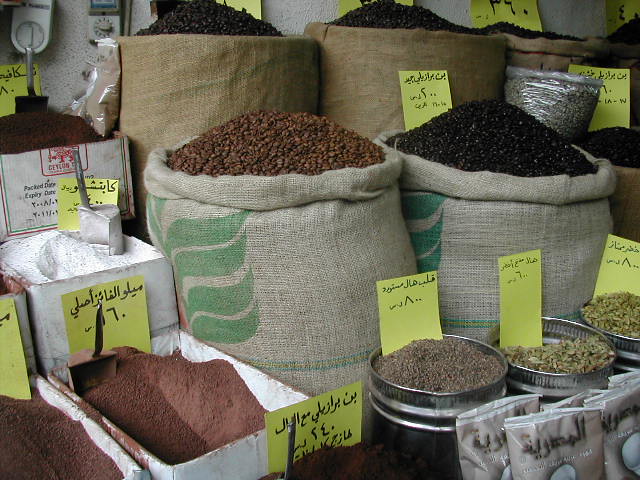The image depicts a vibrant market stall, likely in an oriental setting, brimming with a variety of goods displayed in an organized manner. In the background, against a white wall adorned with a thermostat, a timer, and several sticky notes inscribed with Arabic writing, there are six burlap bags filled with dark brown beans or possibly coffee beans. The bags are uniform in size, except for the one on the far left which is slightly shorter with a metallic cover on top. Notably, the middle burlap bag among these has a yellow sticky note affixed to it.

In the foreground, three more bags are present. The one on the far right contains darker beans, while the middle one shelters lighter brown beans. To the left of these bags is a wooden box filled with flour with a scoop embedded in it.

Further enhancing the layout, three round metal tins filled with light brown, greenish-brown grains or seeds are positioned prominently; each tin has a yellow sticky note with Arabic text. Nearby, two cardboard boxes contain light brown powder, each also marked with a yellow sticky note.

Finally, peeking from the lower right-hand corner of the frame, there are partially visible sealed bags resembling coffee packages, adding to the assortment of goods in this bustling market scene.